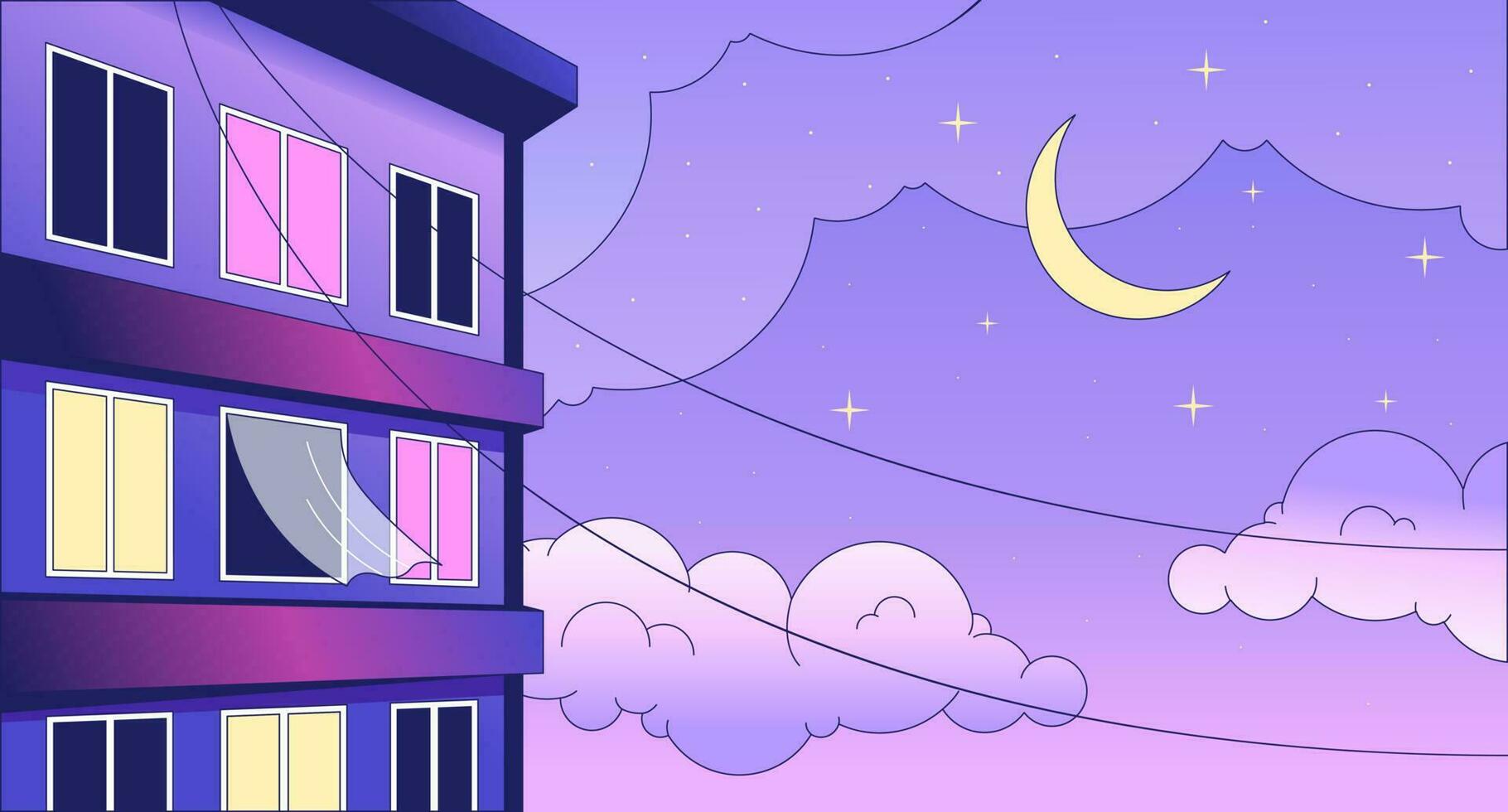This digital illustration captures a night scene featuring the top three floors of a three-story apartment building on the left side. The building is depicted in tones of dark purple and blue, reminiscent of the pastel palette used in the Steven Universe series. Each floor features three windows, with a mix of illuminated hues—some in yellow, some in pink, and some in light blue, with one window notably having a curtain floating outside. The sky forms an exquisite ombre backdrop transitioning from lilac to light purpley-pink, dotted with black-outlined clouds of light purple, blue, and white. Central to the sky is a yellow crescent moon accompanied by small yellow stars. Two diagonal lines, possibly representing power lines, extend from the top of the building across to the bottom right of the image. The clarity and brightness of the illustration are enhanced by the distinct lighting and vivid color contrasts, making the night setting pop with vibrancy.